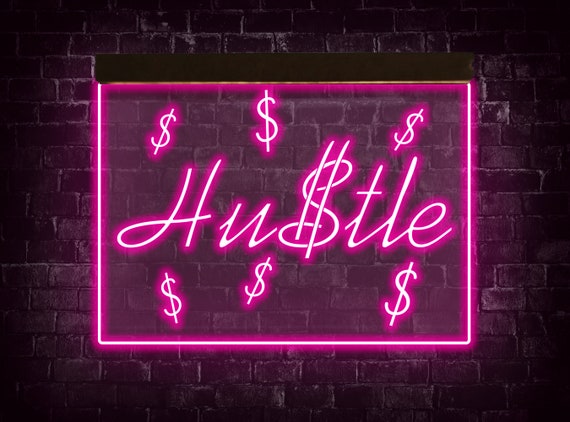The image features a rectangular neon pink sign that prominently displays the word "Hustle" in a cursive font, with the 'S' cleverly stylized as a dollar sign. Surrounding the word "Hustle" are six smaller dollar signs, arranged with three at the top and three at the bottom. The neon tubing emits a vivid pink light, with the center of the sign almost appearing to be see-through, adding an ethereal glow to the frame. This vibrant sign is set against a dark brick wall, which suggests the setting could be industrial or urban. The bricks are standard-sized and the overall lighting is dim, making the neon sign the focal point. It’s challenging to discern whether the sign is mounted on the wall or floating in front of it. Additionally, the edges of the image fade into black, enhancing the dramatic effect and ensuring that the neon sign stands out. Some vague assemblies at the top of the sign indicate the presence of electronic components.